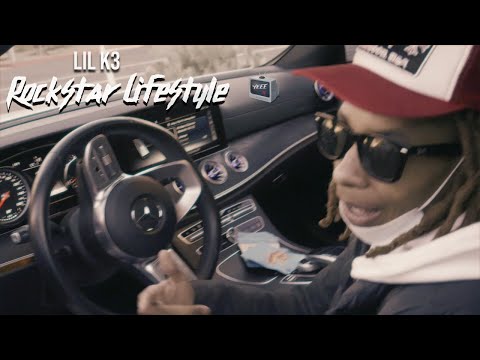In the image, a young African-American man with light skin and brown dreadlocks is seated inside a black-interior Mercedes-Benz car. He wears a red and white trucker-style cap and black sunglasses, and has a white medical mask pulled down to his chin, revealing his open mouth as if in mid-conversation. The man, dressed in a black top, is gesturing with one hand toward something or someone outside the driver's side window. The car's steering wheel prominently displays the Mercedes-Benz logo, and the dashboard, including a speedometer with a red needle and white markings, is clearly visible. Through the windshield, a brown-hued scene unfolds. The photograph, rectangular in shape and bordered by thick black lines at the top and bottom, features the white text "Lil K3 Rockstar Lifestyle" positioned at the top left corner.